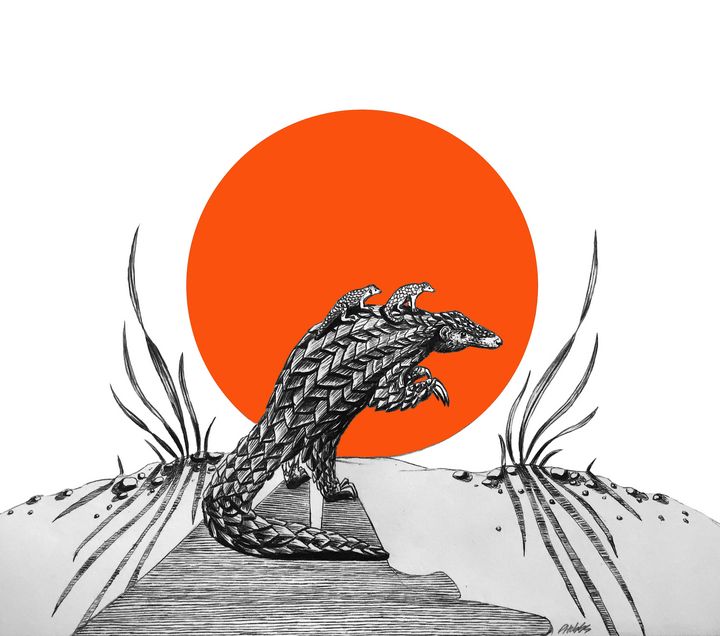The artwork is a detailed black-and-white drawing of an armadillo standing upright on its hind legs. Positioned on the armadillo's back are two smaller armadillos, likely its babies, mirroring the adult's posture by also looking to the right. The scene is set against a stark background dominated by a large, round orange circle that likely symbolizes the Sun, casting the armadillo's shadow behind it. The ground beneath the armadillo appears to be sandy or rocky, adorned with scattered rocks, pebbles, and some small plants on both sides. The artist's signature can be found at the bottom right near the shadow.